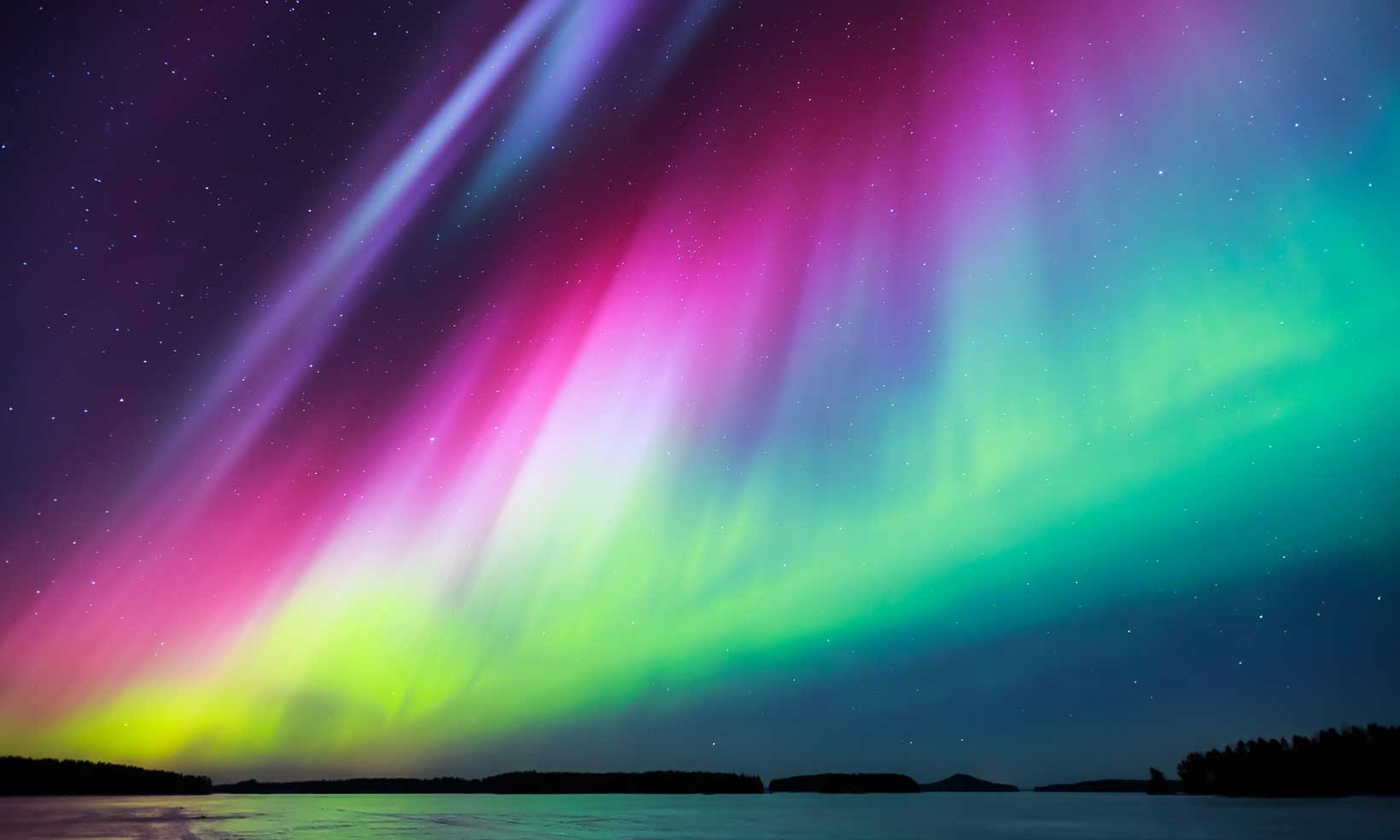In this captivating nighttime image, a stunning aurora borealis, or northern lights, illuminates the sky over a serene body of water, likely a lake or pond, surrounded by a distant dark tree line. The mesmerizing light show stretches across the entire sky, starting with a deep purple at the top, gradually blending into bright magenta, transitioning to lighter violet, pink, and navy blue hues, before evolving into vibrant strips of green and yellow. Small stars dot the sky, twinkling through the array of colors. Whether an actual photograph or a masterful computer-generated image, the scene beautifully captures the dazzling interplay of colors characteristic of the northern lights, creating a breathtaking celestial display.